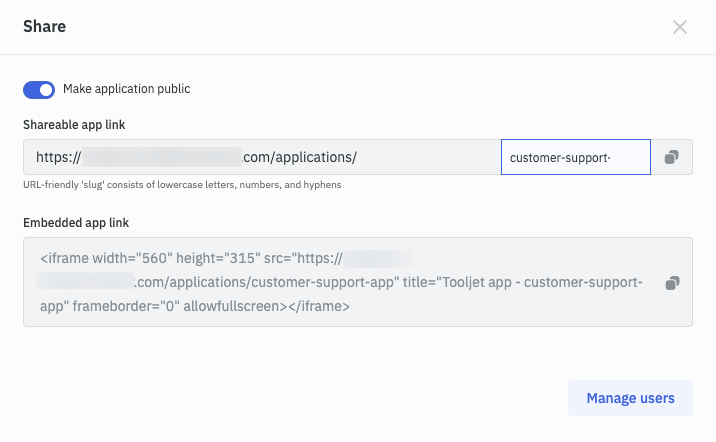The image features a clean, white background. At the top left corner, the word "Share" is displayed in black text. On the far right, there's a faint gray "X." Just below, a thin gray line stretches from the left to right edge of the image. Underneath this line, the phrase "Make application public" is prominently displayed in black text. Adjacent to this text is a blue toggle switch, which is positioned to the right, indicating that it is turned on.

Below this section, the phrase "Shareable app link" is written in black. Beneath it, there's a banner that resembles a search bar. In this bar, a URL is partially visible, starting with "https://" and continuing with some portions whited out. The visible part of the URL reads "com/application/". On the right side of this banner, a smaller white banner outlined in blue contains the text "Customer Support" in black. Adjacent to this, there are two small square icons.

Further down, a segment explains that a "URL-friendly slug" should consist of lowercase letters, numbers, and hyphens. 

Next, the section labeled "Embedded app link" in black features a large light gray box filling the width of the image. Inside this box, the text starts with "<iframe width="560" height="315" src=", followed by a partially visible whited-out URL starting with "https://" and ending with "com/application/customer-support". It continues with 'title="Tool Jet App - Customer Support" app', followed by 'frameborder="0" allowfullscreen></iframe>'.

Beneath this shaded box, there's a white space. In the right corner of this space, a small shaded banner with the text "Manage users" is written in blue letters.